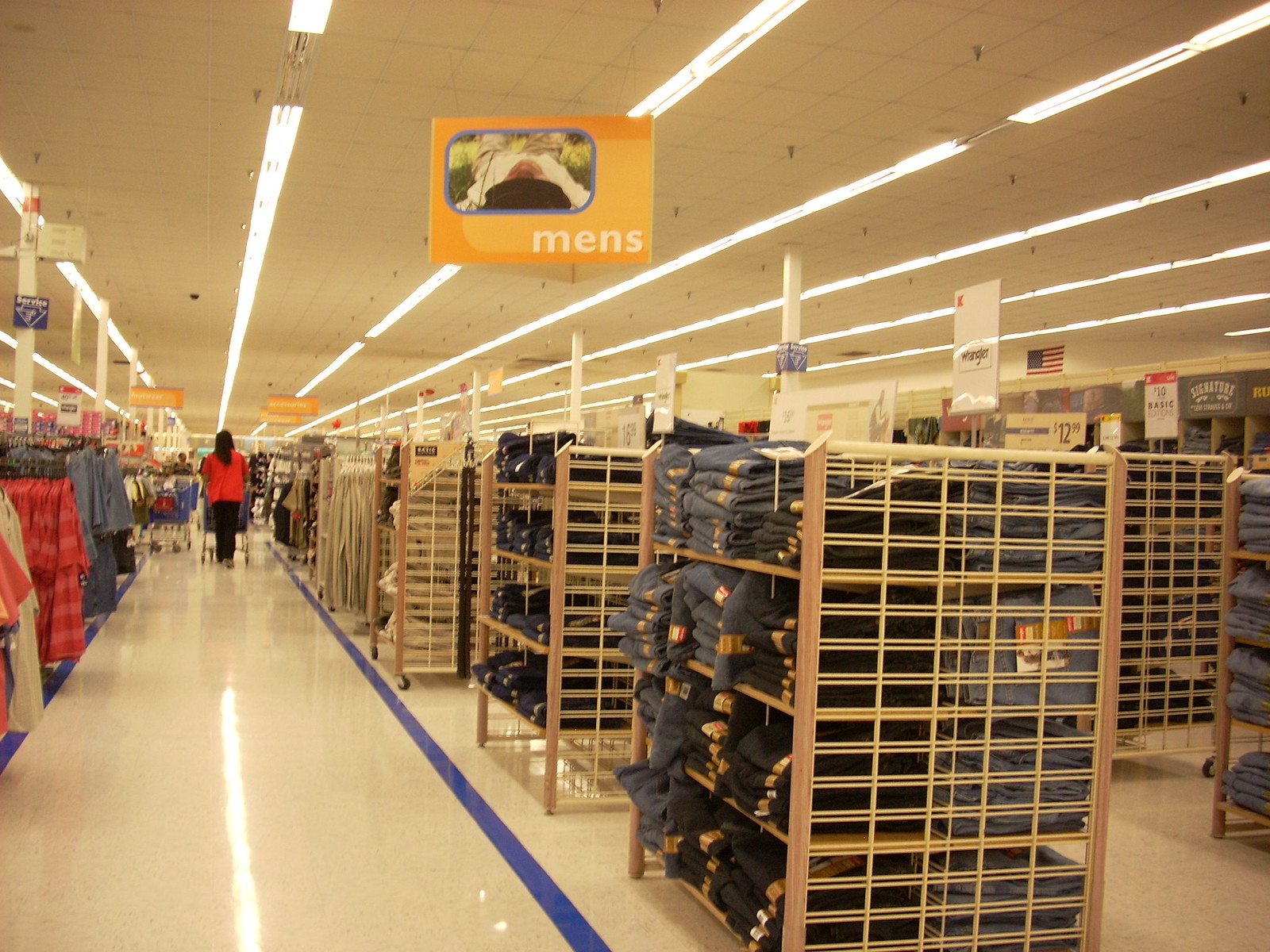The image captures the men's department in a department store teeming with a variety of clothing items and bustling activity. At the very forefront stands a light wooden rack with four shelves, each densely stacked with jeans. To the right of this rack, additional similar wooden racks also brimming with jeans can be observed. On the left, a walking path meanders through the store, guiding the viewer's eyes down a corridor lined with even more racks of jeans. 

Further along this path, a hanging rack displaying an assortment of khaki pants comes into view. Adding to the scene's dynamism, a lady dressed in a red shirt and black pants is seen pushing a shopping cart away from the viewer. Close by, another shopper maneuvers a cart toward the viewer, navigating through the aisles. 

To the left of this approaching cart, various hanging clothes are organized, including racks of gray shorts, red shirts, and tan shirts. Crowning the top of the image is an orange sign emblazoned with the word "Men's," featuring an illustration of a man reclining. The ceiling is illuminated by long strips of lights, casting a bright and inviting glow over the department.